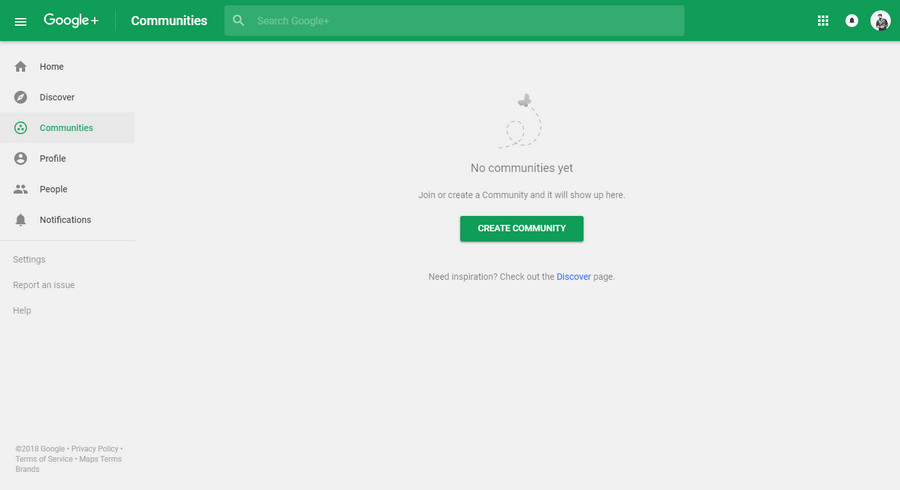Screenshot of a Google+ Communities page interface. At the top, a green bar spans the width of the screen. On the upper left side of this bar, the white text "Google+" is prominent. To the right of this, the word "Communities" can be seen, followed by a search bar containing placeholder text reading "Search Google+." On the far right of this bar, a small white circle contains the profile picture of a man.

The background of the page is a light gray. On the left side, there's a navigation panel with "Communities" selected, highlighted by a icon resembling a circle with three dots arranged in a triangular pattern. In the main content area, towards the top, a butterfly icon is displayed. Below this, text reads "No communities yet. Join or create a community, and it will show up here."

Centered on the page, a large green rectangle contains the white text "Create community." Below this button, smaller text prompts users with, "Need inspiration? Check out the discover page," where the word "discover" is highlighted in blue, indicating a clickable link.

In the bottom left corner of the page, footer text provides links to "2018 Google," "Privacy Policy," "Terms of Service," "Maps Terms," and "Brands."